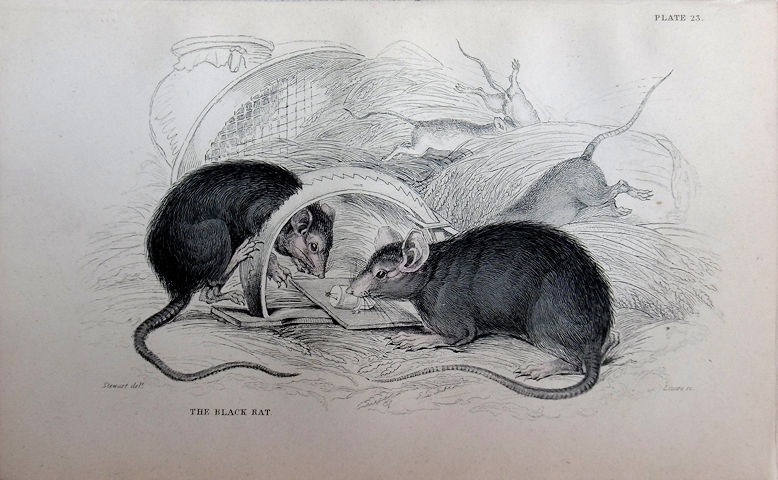This is a masterfully detailed black and white pencil drawing titled "The Black Rat," labeled as plate 23. The artwork captures a scene teeming with black rats set against a background of strewn objects, hay, straw, and natural grasses. In the foreground, a mousetrap has snapped shut, ensnaring one rat's head and front feet, while another rat cautiously investigates the trap. Two highly detailed rats dominate the scene, their profiles showcasing full bodies covered in black fur, long ribbed tails, short legs, elongated feet with light gray toes, and large upright ears. The background features three additional, more muted rats in gray and nearly white tones: one with its feet and tail visible, another appearing to run through the hay, and the third partially hidden. Piles of hay and an indistinct jar further set the scene, enhancing the natural and somewhat chaotic environment. The artist’s name appears, though it remains unreadable, firmly grounding the piece as a blend of scientific intricacy and artistic expression.